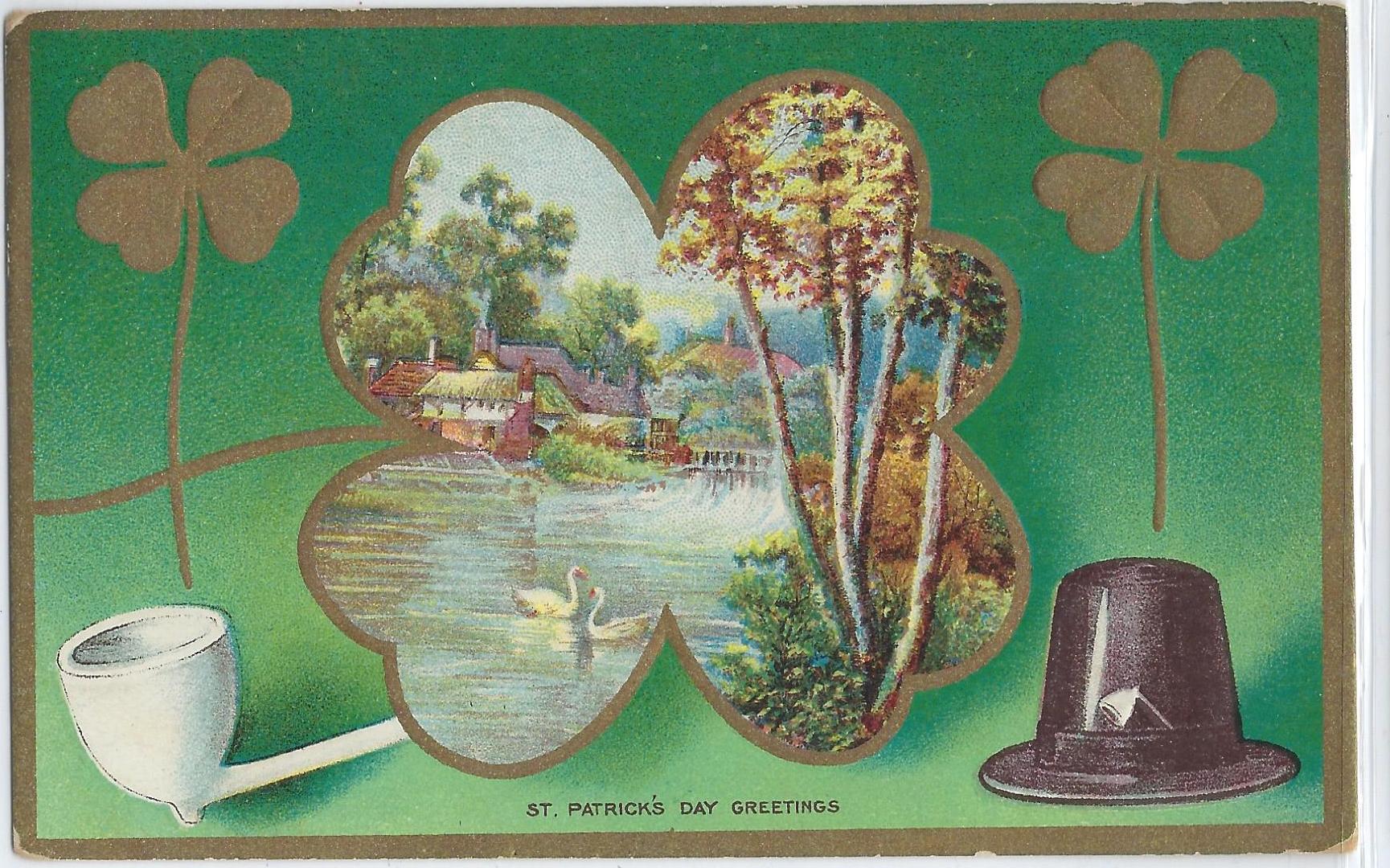This vintage St. Patrick's Day greeting card features a gradient green background with slightly weathered corners, framed by a gold border. At the corners of the card are two imprinted brown four-leaf clovers. Dominating the center is a large four-leaf clover with a gold outline, enclosing a picturesque painting. The painting depicts a serene scene with swans swimming in a lake, surrounded by trees adorned with yellow and red flowers and thin trunks. In the distance, a quaint village with various houses, including a red-roofed building and a thatched hut, adds to the rustic charm. A subtle waterfall or dam is visible to the right of the lake. On the bottom left of the card, a white smoker’s pipe is featured, while a black pilgrim-style hat with a pipe sticking out adorns the bottom right. The text "St. Patrick's Day Greetings" is elegantly inscribed at the bottom of the card, adding a festive touch.